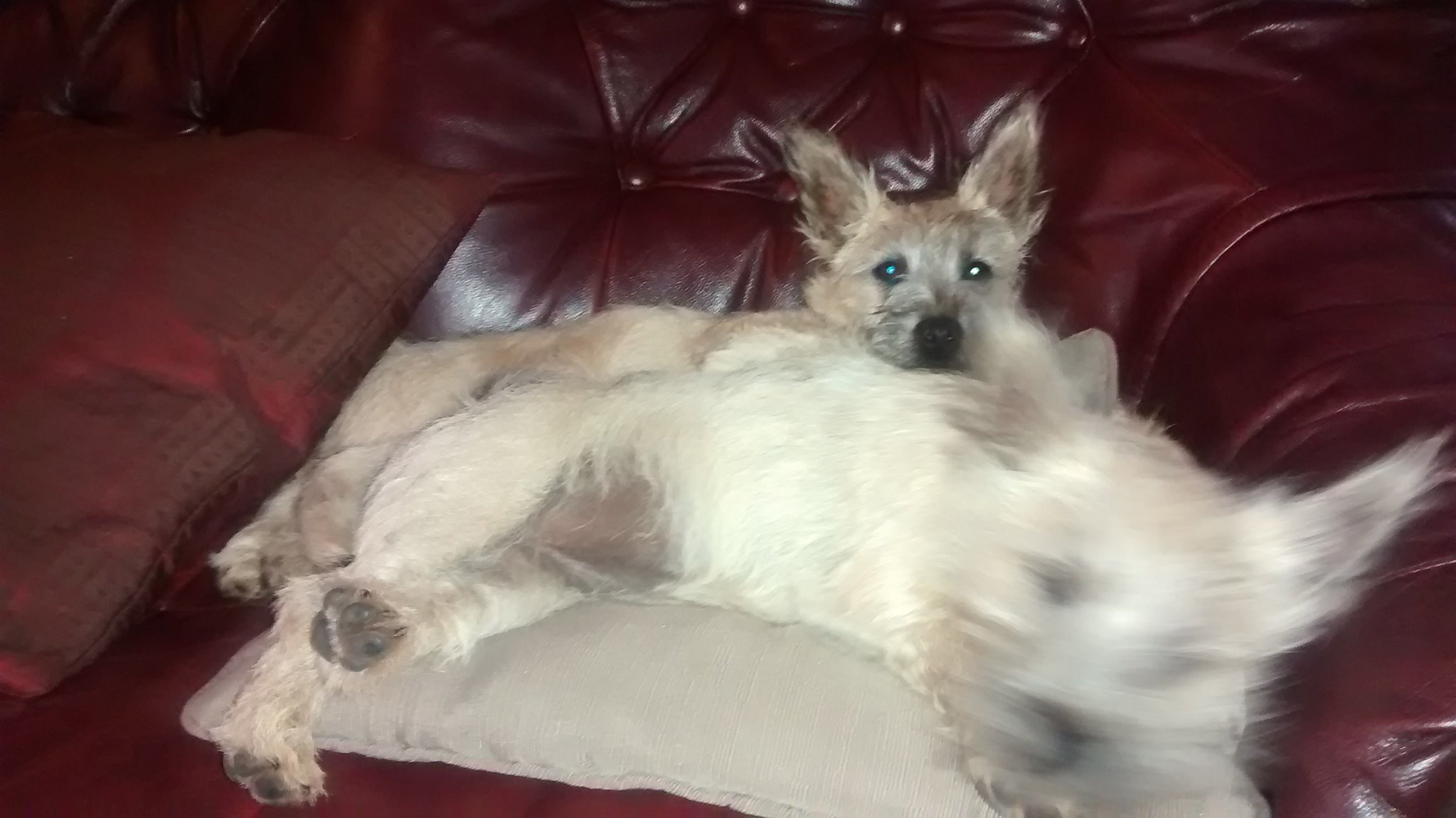In the image, two white, furry dogs of similar size and build are comfortably nestled together on a luxurious red leather couch. Surrounding them are matching red pillows, enhancing the cozy ambiance. The focal point is a cream-white pillow on which both dogs are positioned. One of the dogs appears calm and relaxed, laying down peacefully, while the other seems to be in the process of getting up, suggesting a moment of playful activity or curiosity. Their close proximity and similar appearances suggest a bond or relationship, adding a heartwarming element to the scene.